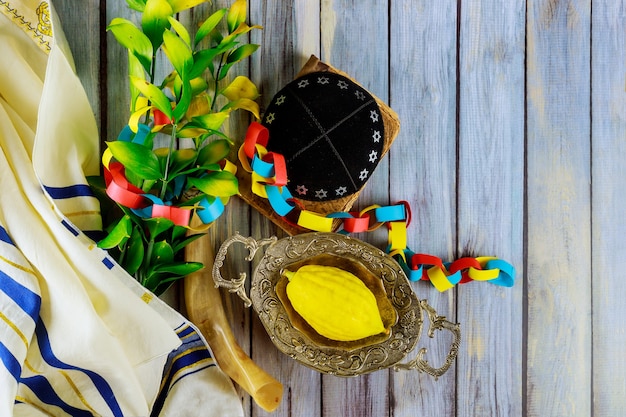The photograph captures a collection of assorted objects artistically arranged on a wooden surface with visible black slots between the planks. The wooden surface, grey with white spots, might be a floor or table. Central to the image is an ornate bowl with two handles, featuring elaborate etching around its edge. This bowl, appearing to be brass or copper but likely plastic, contains a vividly yellow toy lemon. To the left of the bowl lies a white cloth or shawl adorned with blue and thin gold stripes. Adjacent to this is a bouquet of shiny, plastic-looking leaves with light green stems and green leaves tipped with yellow, mimicking blossoms. A colorful chain of paper links in blue, red, and yellow hues loops around these objects, snaking through a horn, the bouquet, and onto the wooden surface. The ensemble is further adorned by what seems to be the black cover of a jar peeking into the frame from above.